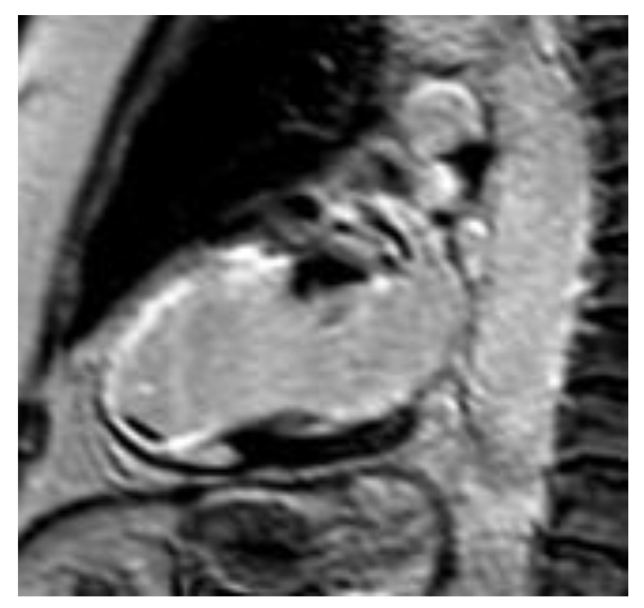The image is an extremely low-quality, grayscale scan, so blurry and grainy that discerning details is quite challenging. Dominated by a solid black background, the central portion showcases a large light gray blob, which might be assumed to represent a part of a medical scan due to its ambiguous and textured appearance. This central blob is flanked by other, smaller gray blobs to its left and right, and directly below it resides a darker gray oval shape. In this hazy expanse, there's an indistinct feature—resembling an upside-down face or skull—evoking comparisons to either a grainy moon crater photo or part of an anatomical scan. One interpretation suggests it might be the footprint of a fetus depicted in a sonogram, with three distinctive toes angled diagonally, adding a faint, almost cartoonish charm amidst the nebulous shapes.